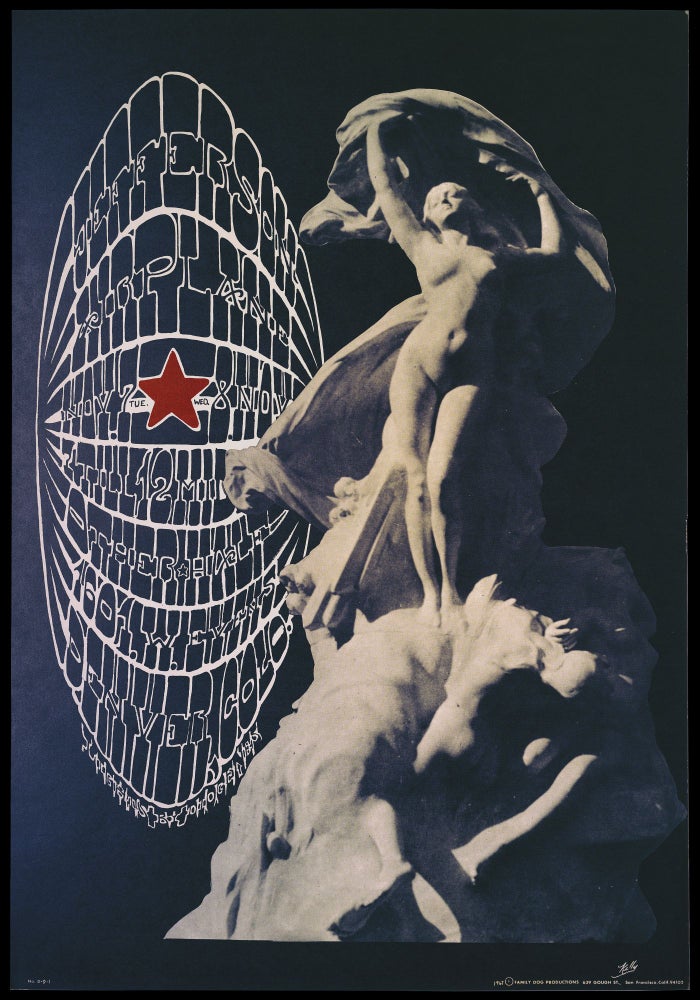This is a highly abstract and visually striking poster with a very dark navy blue background dominated by two primary elements. On the left side, intricate and harsh white lines bend and curve dramatically, creating a warped perspective as if being pulled forward, with both vertical and horizontal lines converging towards a central red five-point star. These lines, seemingly forming a distorted text, are challenging to decipher but appear to state "Denver cold" at the bottom. The right side of the poster features a monochromatic photograph of a marble statue of a naked woman. She is portrayed in a dynamic pose, holding a flowing piece of fabric above her head with her left hip jutted out. The statue, detailed with shadows and highlights, stands atop an ambiguous form, possibly a rock face or mound, and is enveloped in partial shadow that accentuates her contours. The overall color scheme of the poster comprises black, white, and red, contributing to its bold and compelling visual impact.